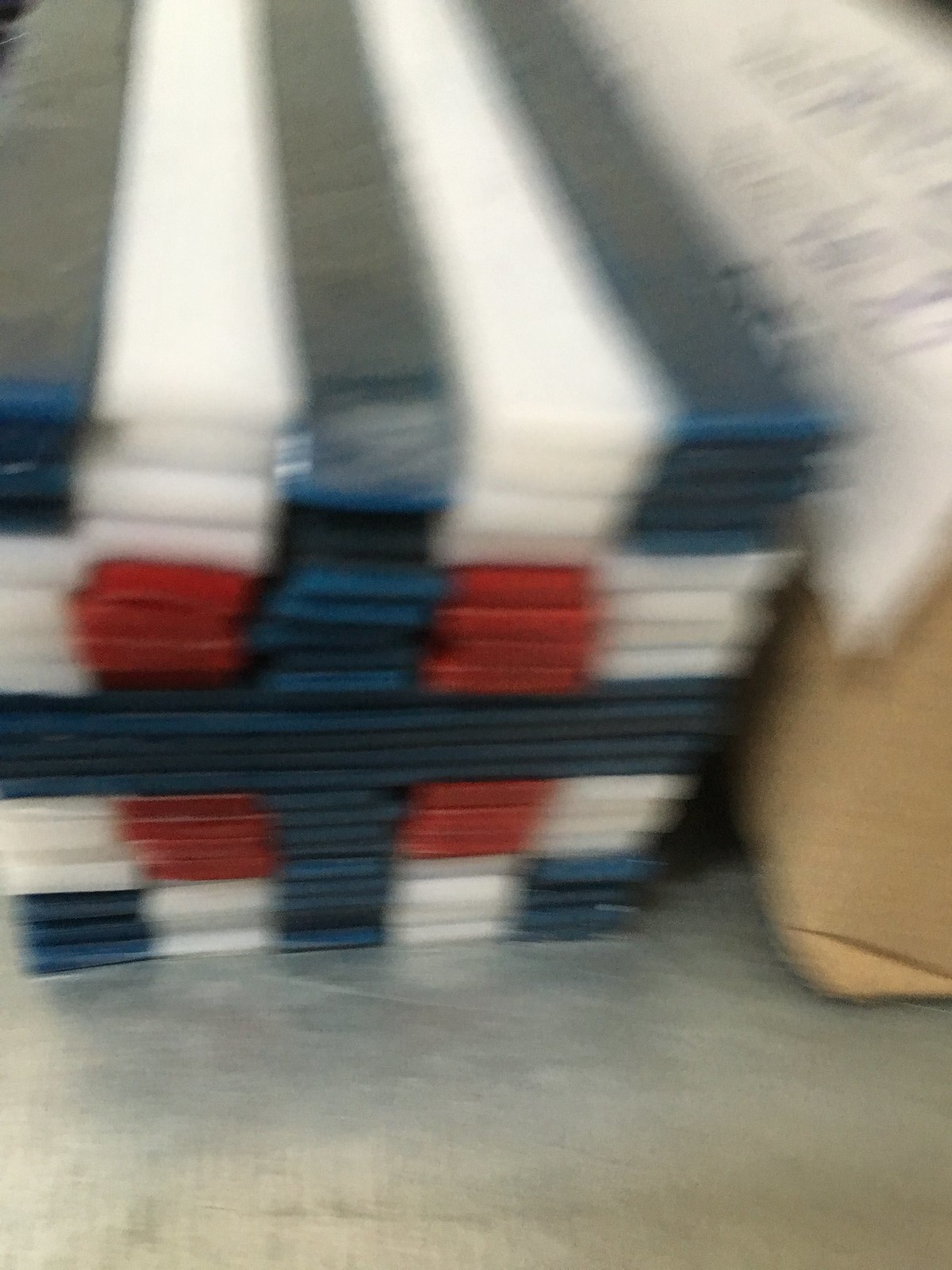The blurry close-up image shows a stack of multi-colored fabrics, possibly curtains or bed sheets, neatly arranged into a rectangular shape. The fabrics are organized in various layers, each consisting of rows of four, with colors meticulously alternating. At the top, the stack begins with gray fabric featuring blue accents, followed by alternating layers of white and gray. Subsequent layers include patterns of white, red, and blue fabrics. The fabrics are both horizontally and vertically stacked in sequences of colors including dark blue, light blue, and red. The background reveals a light gray floor with dark gray sloshes, and a large cardboard box containing white materials on the right side of the image. Despite the photo's blurriness, the vibrant colors and structured arrangement of the fabrics are evident.